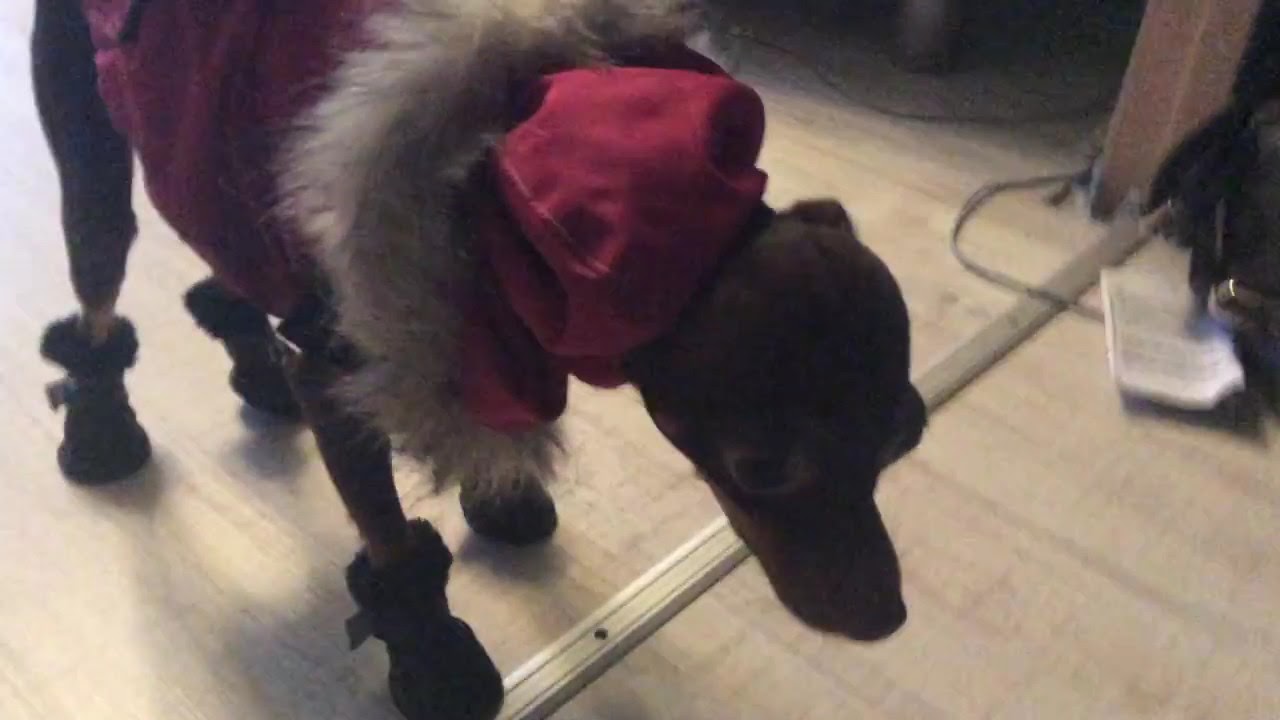The image is an indoor photograph featuring a small brown dog, likely a Chihuahua, wearing a red coat with whitish fur trim around the neck and black little booties on each paw. The dog has a downcast expression, appearing somewhat sad or uncomfortable. It is standing on a tan-colored hardwood floor beside a small metal doorframe. In the upper right corner of the image, there are a few pieces of white paper with black writing, positioned near a trash bin. Additionally, a black or dark brown wire is visible on the floor, and the overall quality of the photo is somewhat low, with a bit of a grainy and blurry effect.